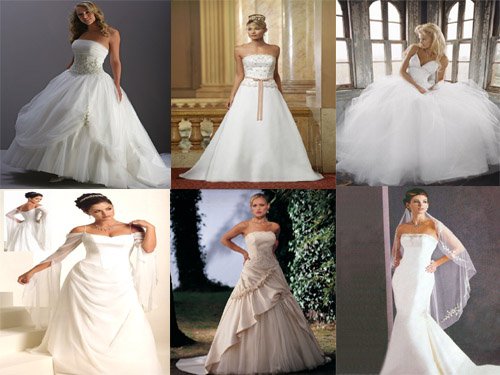This image is a composite showcasing six different bridal gowns worn by models with fair to medium skin tones and predominantly brown or blonde hair. The layout features three gowns on the top row and three on the bottom, each set against distinct backgrounds. 

1. **Upper Left**: This gown is strapless with a full ballgown-style skirt. The blonde model stands against a gray background with her hair thoughtfully curled, embodying a classic, princess-like look.
2. **Upper Middle**: This strapless gown features an A-line skirt with a pink ribbon belt. The model, with her hair elegantly styled in a bun, poses in front of a grand, castle-like backdrop with beige pillars and railings, adding a touch of historical romance.
3. **Upper Right**: The blond model wears a strapless dress with a deep V-cut bodice and a puffy tulle skirt. She poses in front of a windowed, wooden structure, giving a quaint, rustic feel.
4. **Lower Left**: A brunette model showcases an off-the-shoulder gown with bracelet-length sleeves and a full skirt. Styled with a bun, she poses in a white room with white stairs, highlighting the gown’s intricate ruffling and classic elegance.
5. **Lower Middle**: This gown appears to be a slightly off-white color with diagonal ruffles across the gathered skirt. The blonde model stands outdoors with grass and green foliage in the background, providing a natural, serene setting.
6. **Lower Right**: Completing the collection is a strapless mermaid-style gown. The model with dark hair and a veil stands in front of a gray background, emphasizing the gown’s sleek, form-fitting silhouette that flares below the knees.

This detailed composite blends various gown styles and settings, reflecting diverse bridal aesthetics and environments.